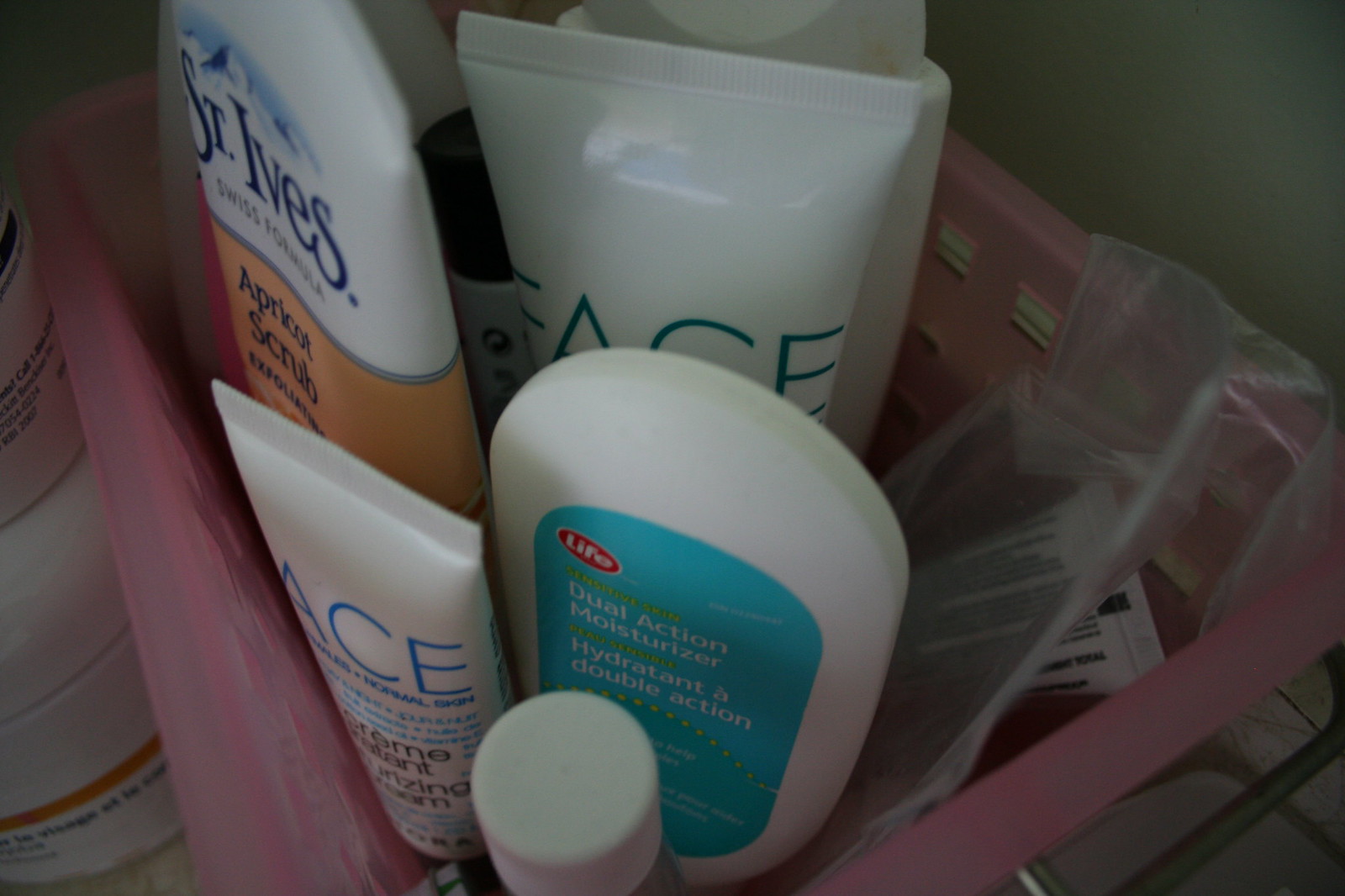This photograph, in landscape orientation, offers a detailed glimpse into a collection of bath products arranged within a plastic pink caddy. The caddy, positioned diagonally from the bottom center to the bottom right of the image, contains various personal care items, giving the impression of a practical and actively used bathroom setup. Prominently visible is a St. Ives Apricot Scrub, identified by its recognizable packaging. Next to it is a product labeled "ACE," whose full name remains unclear. A dual-action moisturizer and a tube marked "face" are also tucked among the items. Additionally, a Ziploc bag contains yet another tube, signifying a careful but utilitarian approach to storage. The overall arrangement of products within the caddy appears vertical, likely to conserve space, and suggests frequent use rather than decorative display. The casual organization underscores the functional reality of an everyday bath routine.